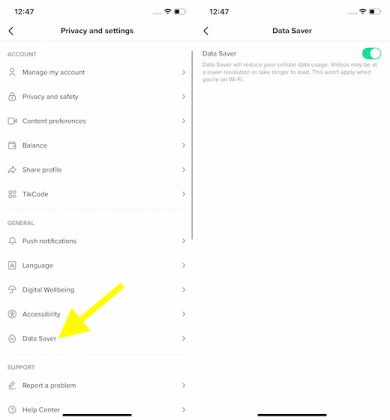The image showcases two side-by-side mobile screenshots, each highlighting different views within a settings menu:

**Left Screenshot:**
- **Top Interface Elements:**
  - Time displayed as "12:47" in black on the top left corner.
  - Wi-Fi signal and battery icons on the top right.
  - Centered title stating "Privacy and Settings" with a left-facing caret on the far left for navigation.

- **Main Settings List:**
  - **Accounts Section:**
    - **Manage My Account:** Profile icon (head and shoulders stick figure).
    - **Privacy and Safety:** Lock icon.
    - **Content Preferences:** Camcorder icon.
    - **Balance:** Wallet icon.
    - **Share Profile:** Right-pointing bubble arrow icon.
    - **HICS Code:** Four-box square icon.

  - A thin, light gray separator line.

  - **General Section:**
    - **Push Notifications:** Bell icon.
    - **Language:** Box with letter "A" icon.
    - **Digital Well-being:** Umbrella icon.
    - **Accessibility:** Star within a circle icon.
    - **Data Saver:** Water drop icon.

  - Another thin, gray separator line.

  - **Support Section:**
    - **Report a Problem:** Pencil writing icon.
    - **Help Center:** Circle with a question mark icon.

  - Each setting entry includes a right-facing caret indicating expandable options.

**Right Screenshot:**
- Replicates the top interface elements from the first screenshot.
- **Data Saver Settings:**
  - Centered title "Data Saver" at the top, again with the time, Wi-Fi, and battery icons.
  - Immediately under the title "Data Saver" on the left.
  - Description: "Data Saver will reduce your cellular data usage. Videos may be at a lower resolution or take longer to load. This won't apply when you're on Wi-Fi."
  - A toggle button to the right of the title, currently switched to the right, indicating that Data Saver is enabled. The toggle's background is green.
  - The rest of the screen below the Data Saver description is blank, filled with white space.

The detailed layout and settings options provide a comprehensive view of the mobile interface for managing account privacy, general settings, and data usage.